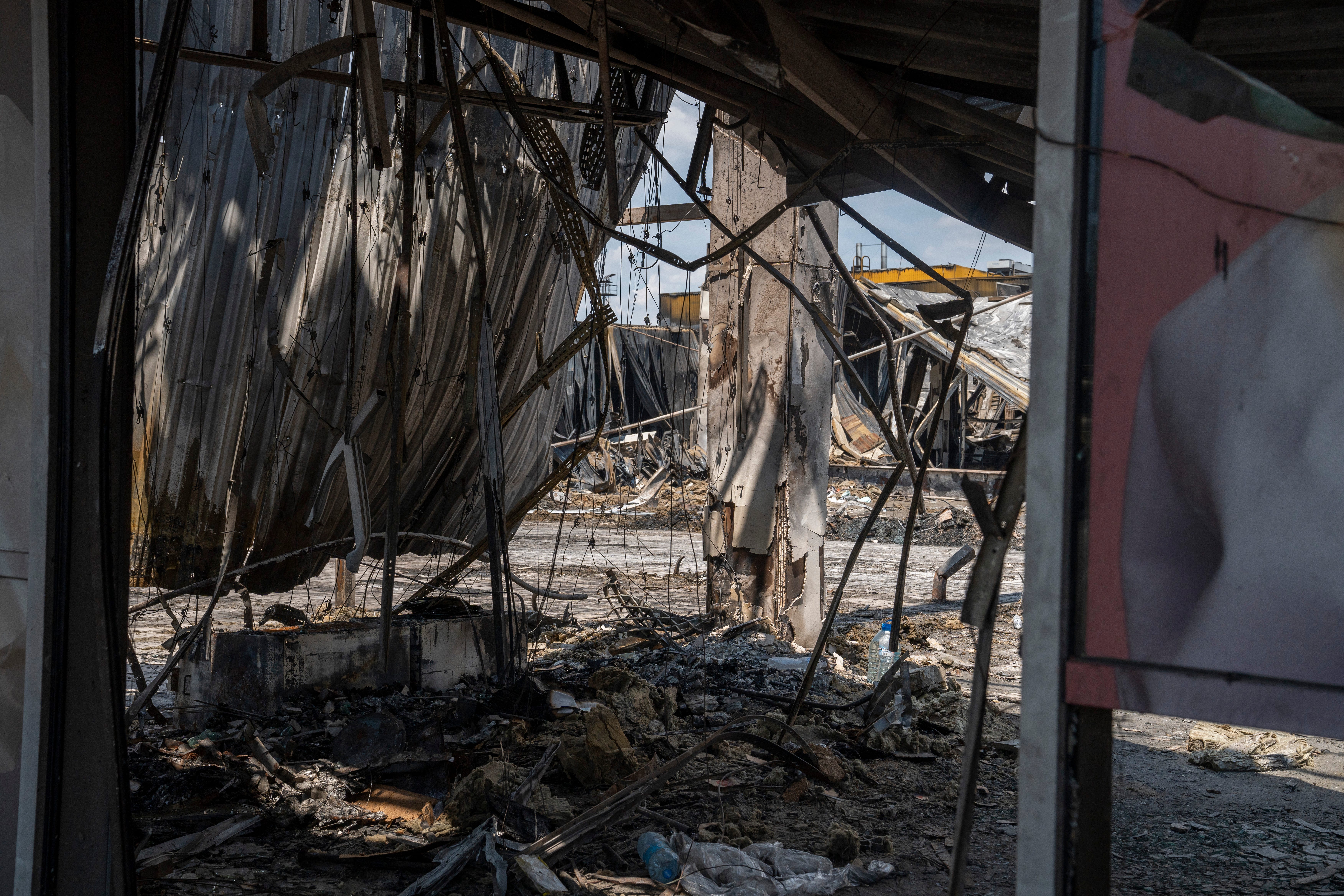The photo depicts a dilapidated or partially demolished building, possibly within a construction zone. The scene is filled with debris, including concrete and dirt, scattered trash, and a twisted assortment of metal and pipes. On the left, a rectangular piece of corrugated tin roofing dangles precariously, and beneath it lies a clutter of rubble. A crumpled sign on a silver pole is visible on the right, flaunting a maroon patch with a silver center and no discernible text. A damaged concrete pillar stands centrally, with its sides peeled away, revealing the interior structure. The floor is littered with rubbish and dirt, hinting at long-term neglect. Another building, seemingly collapsed and tilted, can be seen in the background under a sky dotted with blue patches and some clouds. A yellow construction vehicle is faintly visible amidst the ruins, and several wires dangle from above, enhancing the aura of abandonment.